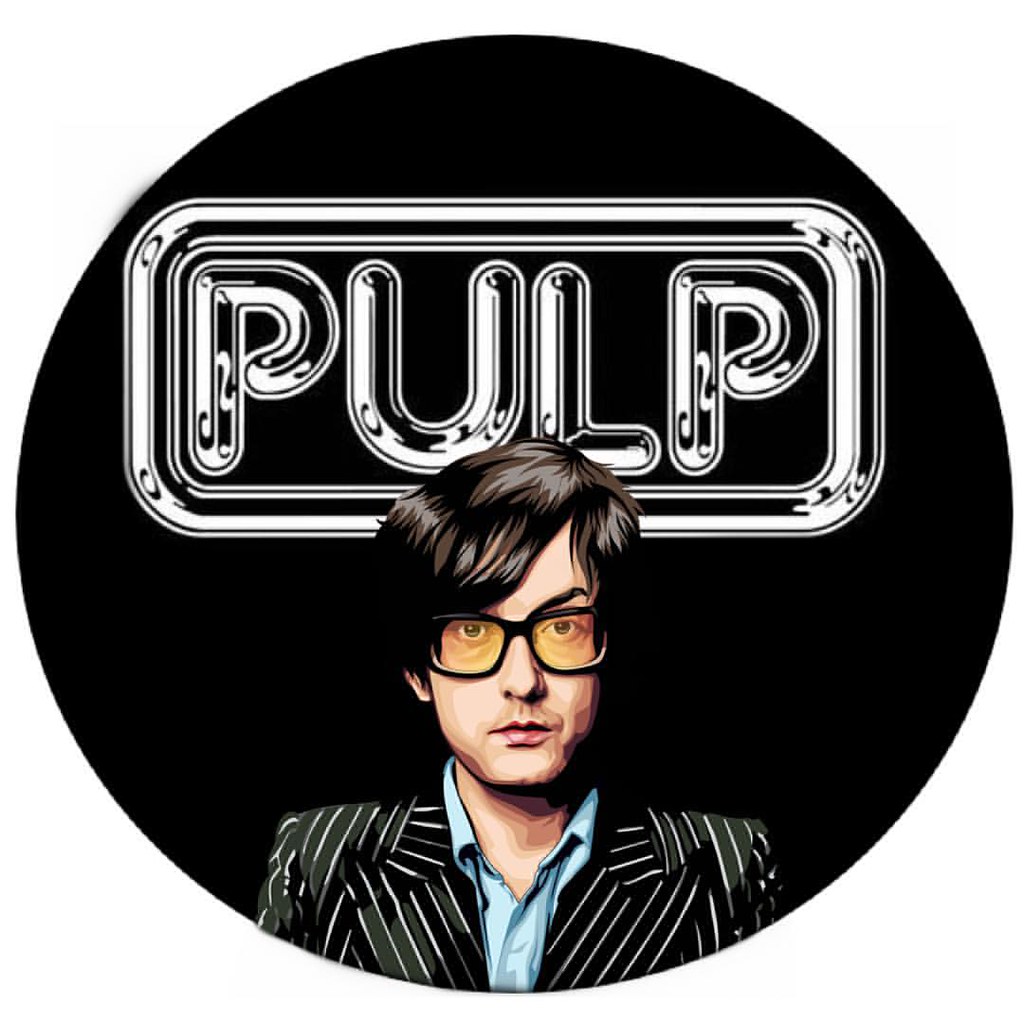The computer-generated image features a stylized portrayal of a Caucasian man standing before a black, circular background. Within this circle is a white, rounded rectangular frame, which contains the word "PULP" in all capital letters. Though reminiscent of neon signs, the sign is unlit, creating a stark contrast against the dark backdrop. 

The man, illuminated in detailed digitization, possesses short, dark brown hair that falls to his ears, with his bangs covering one eyebrow. His visible eyebrow is slightly raised. He sports thick black-framed glasses with a distinctive yellow tint and has a pale complexion, dark eyes, an elongated nose, and red lips.

Dressed in a black and white vertically striped suit jacket over a blue collared shirt, this figure is depicted from the chest upwards, with a neutral expression on his face. The combination of the stylish attire and the graphic elements creates a visually striking and somewhat enigmatic image.